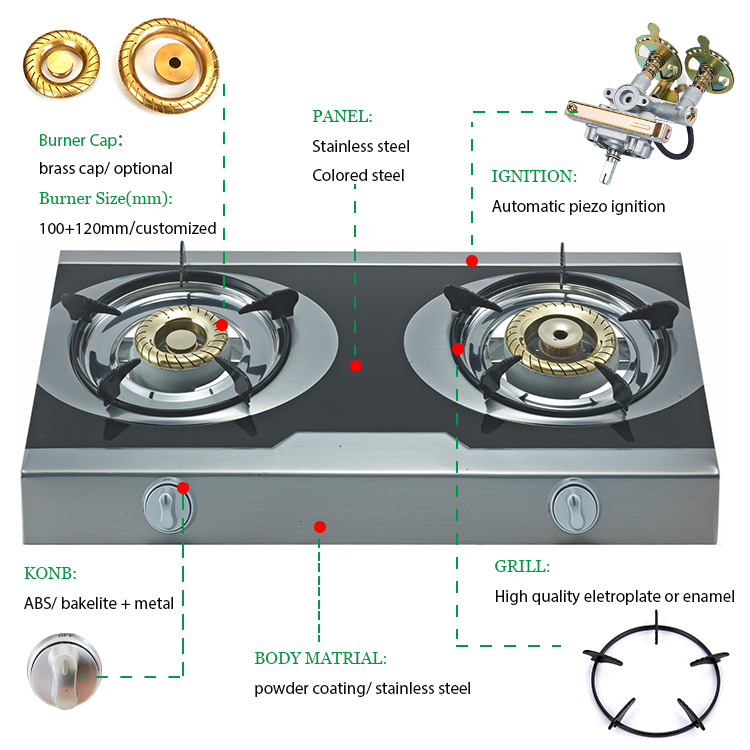The image depicts a detailed diagram of a stove burner, illustrating its internal components and design features. At the center is a dark gray burner, surrounded by silver or light gray elements with brass or gold burner caps, customizable in sizes of 100 mm to 120 mm. The panel is described as being made of stainless steel or colored steel. On the top right corner, the text indicates an automatic piezo ignition system, showcasing two different designs for the ignition. The left side shows labeled parts including the burner cap and sizes. At the bottom, knobs made of ABS Bakelite and metal are mentioned, alongside the body material made from powder-coated stainless steel or high-quality electroplated/enamel finishes. The colors present in the diagram include gold, white, green, black, red, and various shades of gray. This detailed breakdown is likely intended for educational purposes or to assist someone looking to repair or learn about stove burner components.